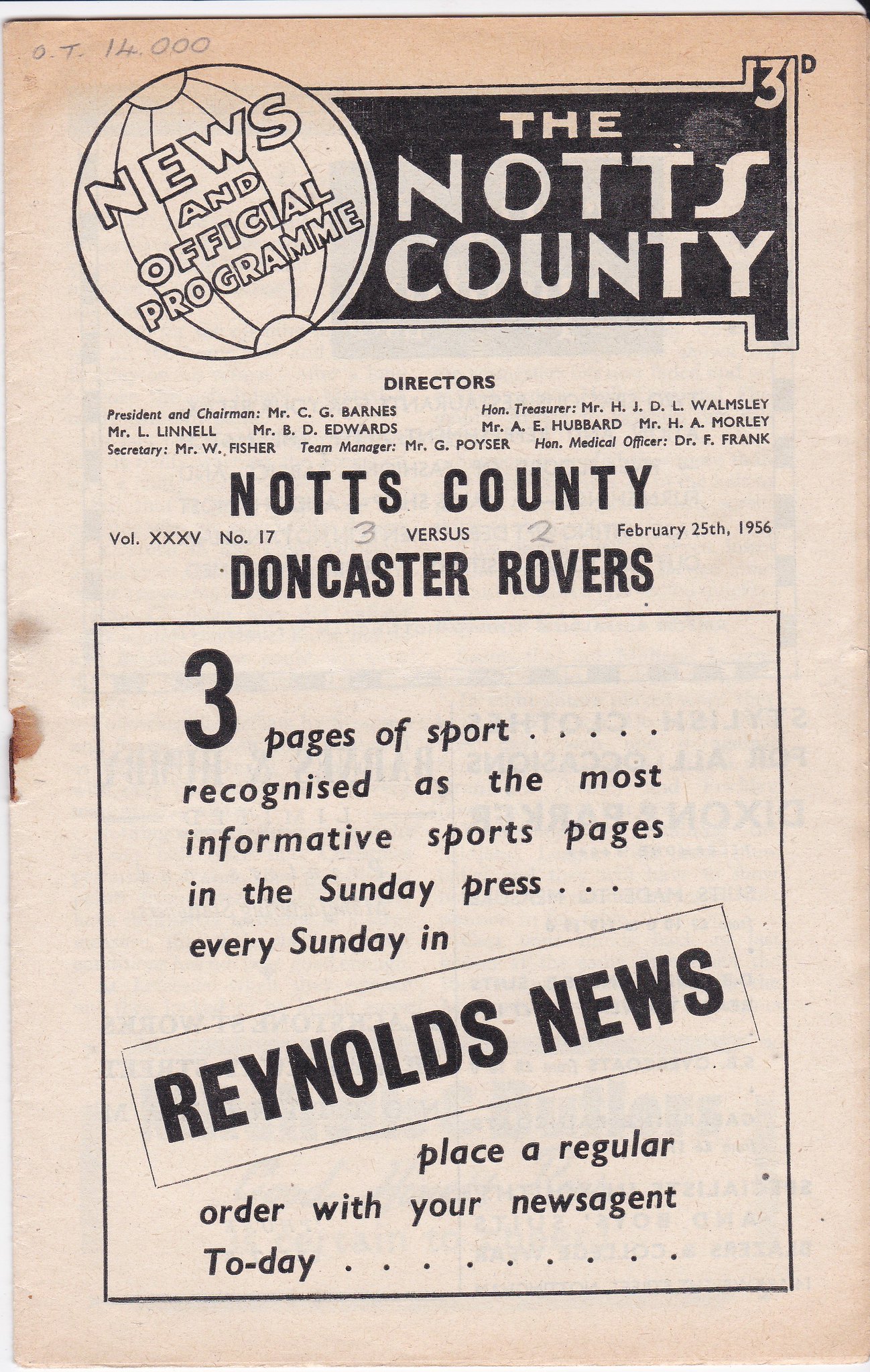The image is an old-fashioned black and white flyer with a light pink background. At the top left, a large circle resembling a globe contains the text "News and Official Program." To the right, "The Knott's County" is displayed prominently within a box. Below, the flyer lists several officials and their titles: Directors and President/Chairman Mr. C. G. Burns, Mr. L. Lionel, and Mr. B. D. Edwards; Secretary Mr. W. Fisher; Team Manager Mr. G. Poizer; Treasurer Mr. H. J. D. L. Walmsley; Honorable Treasurer Mr. A. E. Hubbard; Mr. H. A. Morley; and Medical Officer Dr. F. Frank. Featured prominently in bold font is "Knott's County, Volume XXXV, Number 17, vs February 25, 1956, Doncaster Rovers." The flyer highlights its sports pages as the most informative in the Sunday Press, encouraging readers to place a regular order with their news agent. At the bottom, a white and black square emphasizes "Three pages of sport recognized as the most informative sports pages in the Sunday Press," with "Reynolds News" boldly enclosed in a rectangle at the center. The top left corner also faintly shows the handwritten note "OT14000."